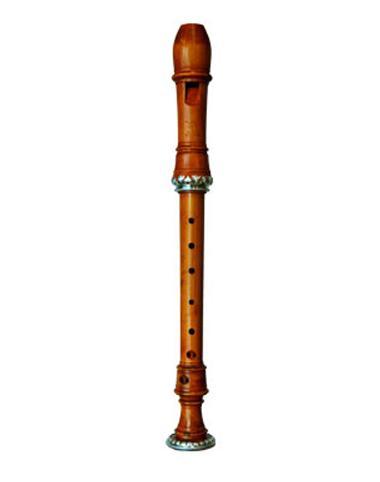The image features a light to medium brown recorder-style woodwind instrument, set against a plain white background. The instrument is upright in the center of the image, with a glossy finish that could be either wood or plastic. At the top is the mouthpiece, which is slightly darker and features a rectangular cut-out with a semi-circular bottom edge. Below the mouthpiece, the instrument widens slightly before narrowing back down, resembling the shape of a salt shaker. Around the top third of the instrument, there is a metallic silver ring that grooves out. There are six finger holes spaced evenly along the central, cylindrical part of the instrument. Toward the bottom, it flares out slightly again, ending in another metallic silver ring.